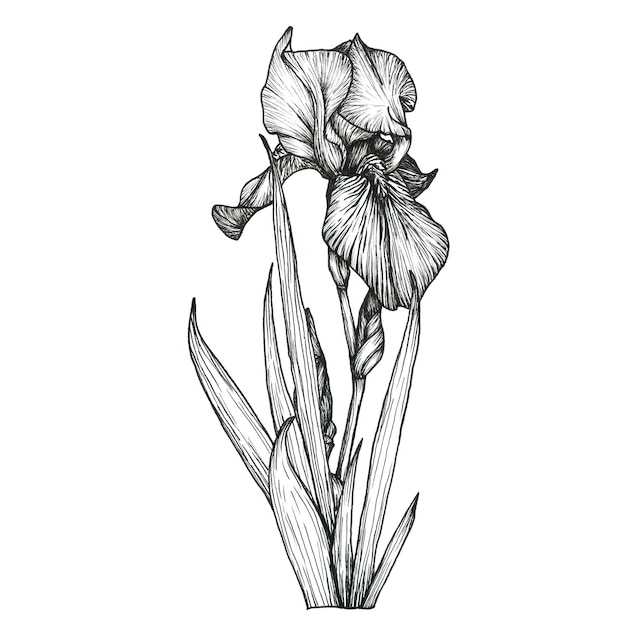This is a black and white pen ink drawing of a flowering plant set against an entirely white background with no framing or text. The plant features long, narrow leaves growing from the ground, which are portrayed as blade-like and detailed with fine lines suggesting subtle texture and ridges. Emerging from the leaves is a central stem that supports a cluster of wispy, fan-shaped petals—resembling shells or elephant's ears. There are around six irregularly positioned petals, with some standing upright and others drooping or facing different directions, giving the flower a natural and dynamic appearance. The illustration is minimalistic, lacking additional elements or colors, which emphasizes the intricate linework and shape of the plant.